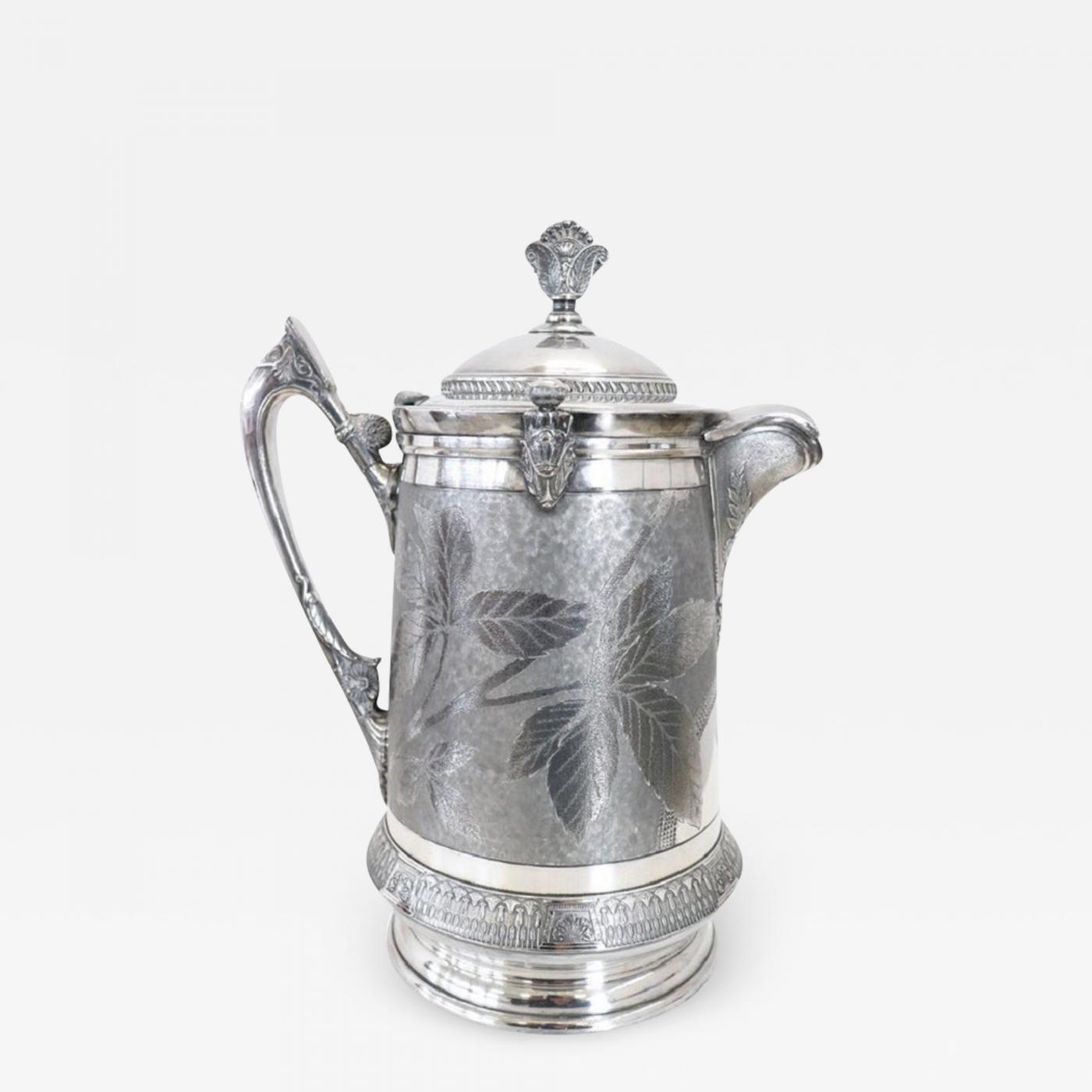The image features an ornate sterling silver kettle or pitcher, beautifully photographed against a completely white background. The kettle's spout is oriented to the right while its elegant silver handle is on the left. The entire kettle has a shiny silver finish, with intricate etchings of leaves around its smoother midsection. Near the base, there's a circular pattern that resembles pearl etchings, contributing to its antique charm. The lid is topped with an ornate and elegant silver knob, adding to the sophistication of the piece. The rim and bottom of the kettle also exhibit a smooth, polished silver design. Overall, this likely early 20th-century antique kettle stands out with its detailed craftsmanship and reflective shine.